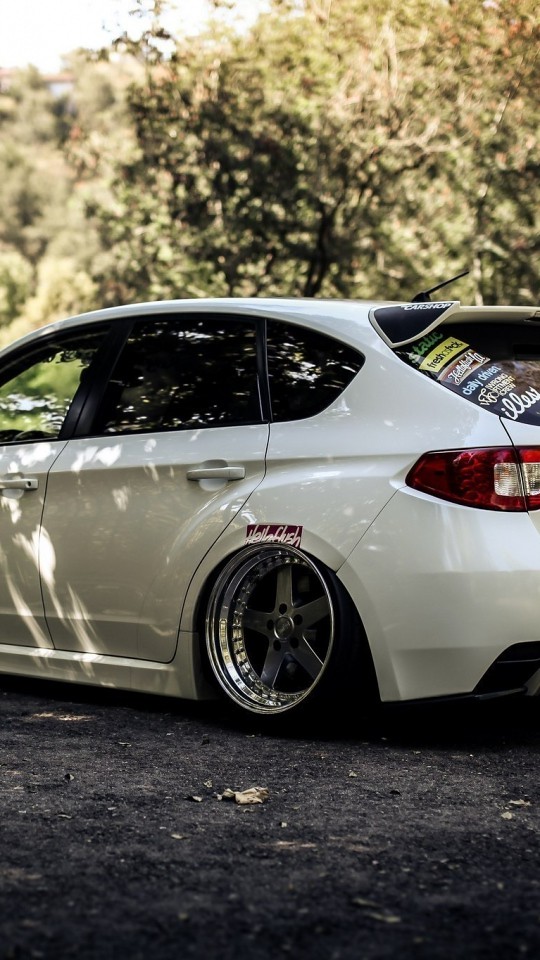The image captures a rear driver's side view of a white Subaru Impreza sedan parked on a rough blacktop or gravel surface, bathed in warm sunlight that filters through nearby trees. The car, known for its sporty and racy modifications, features custom alloy wheels with a prominent Hellfish decal above the rear wheel well. The lowered suspension and slightly cambered wheels further emphasize its drift car style. The rear windows are heavily tinted, obscuring the interior, and adorned with multiple decals. A small fin or fairing sits along the top edge of the rear window, adding to the vehicle's aerodynamic aesthetics. In the blurred background, trees and possibly a hill can be discerned. The overall scene exudes a sense of dynamic stillness, capturing the essence of this modified, performance-oriented Subaru Impreza.